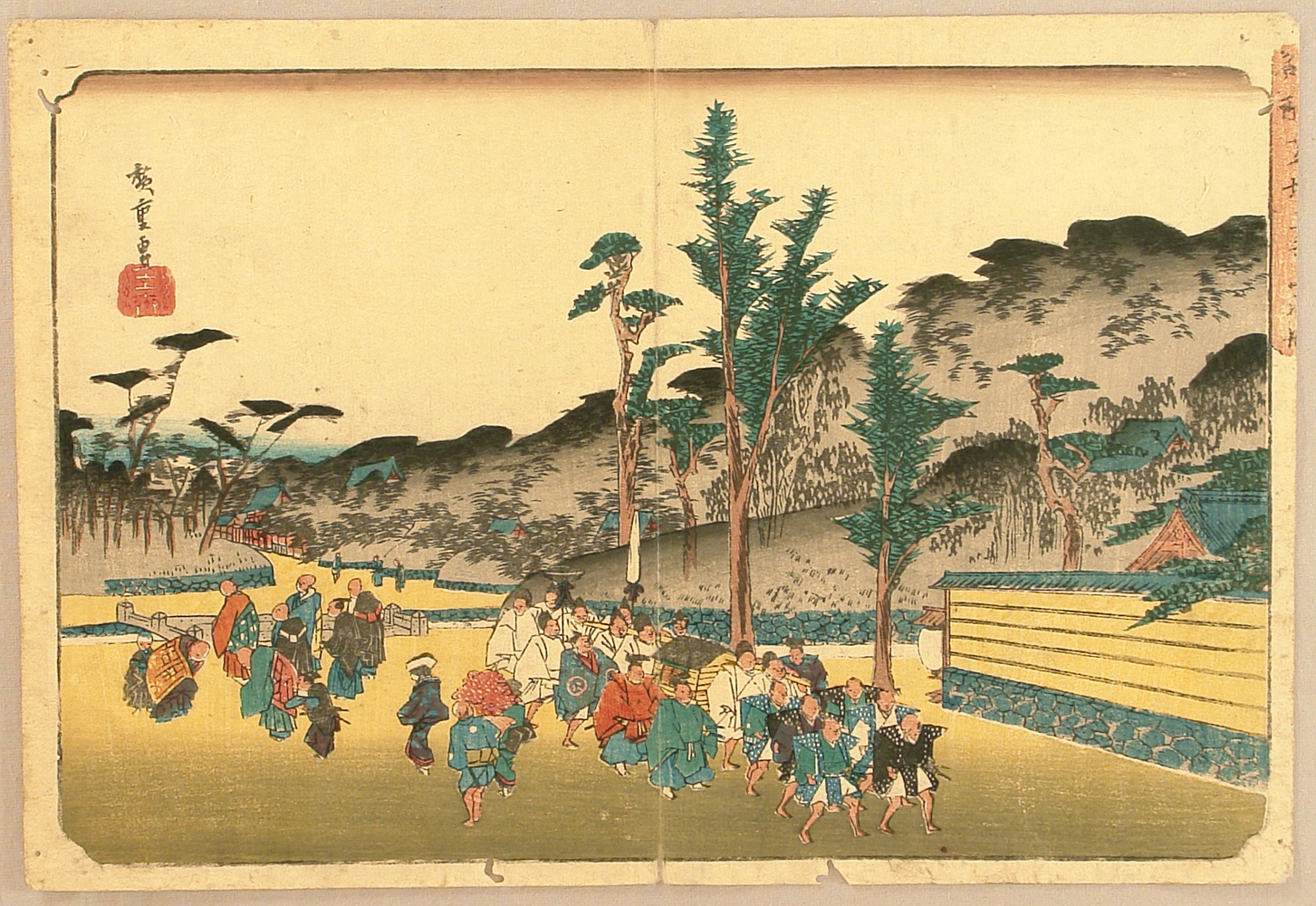This is an image of an ancient piece of Asian artwork, possibly Japanese or Chinese in origin. The detailed painting depicts a traditional and ceremonial scene in a rural village nestled in a valley, framed by mountains on the right and a hillside on the left. In the foreground, a line of people dressed in historical attire are carrying a structure resembling a small wooden house or a ceremonial carriage, possibly used for an emperor or during a funeral ceremony. The men carrying the carriage wear white robes, while others in front are dressed in black and green traditional jackets with large padded shoulders. In contrast, a second group of villagers is shown bowing down in reverence as the carriage passes by. The scene is enriched with additional cultural elements, such as a meandering river that runs through the village field, various trees, and traditional buildings, embodying the quintessence of ancient Asian life and rituals.